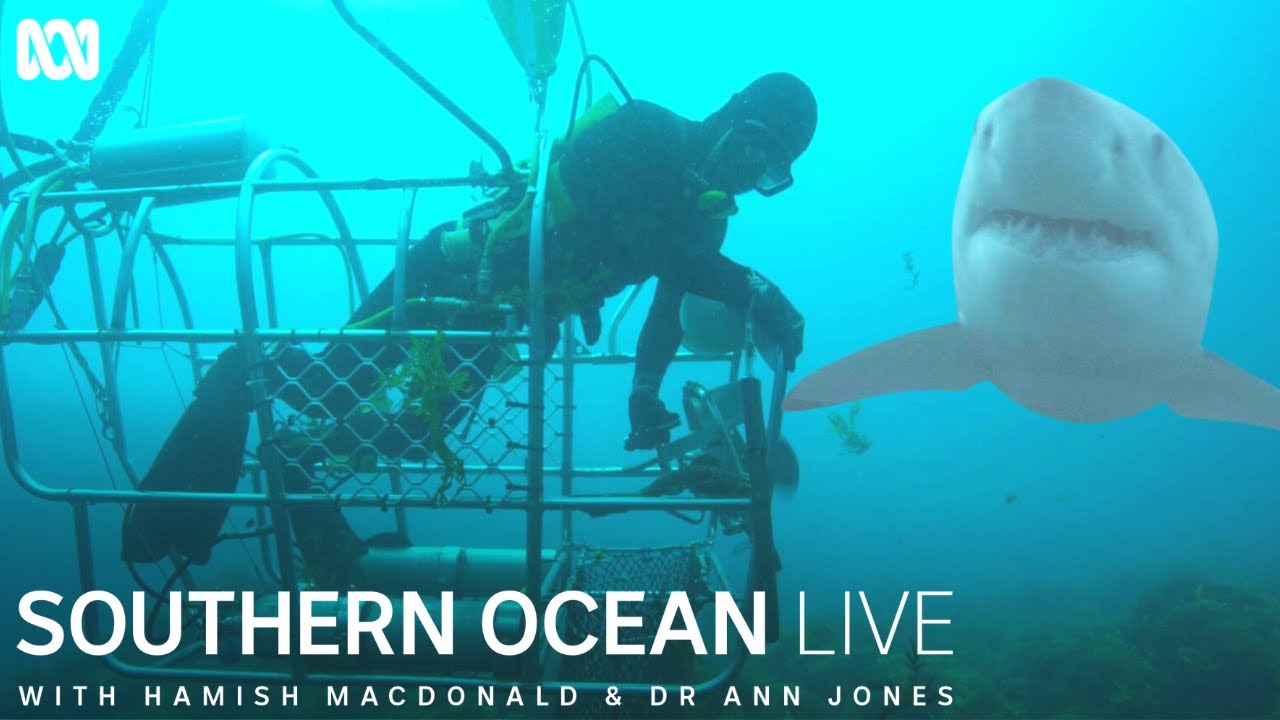This underwater scene captures an intense moment in the Southern Ocean, with divers encased in a metal cage equipped with various instruments. The diver, decked out in full scuba gear—including fins, wetsuit, goggles, and a tank—is suspended in the aqua waters by a cable from an unseen boat above. The gradient background shifts from a bright, lighter aqua at the top to a darker hue at the bottom. Dominating the foreground is a menacing great white shark, its mouth agape to reveal rows of sharp teeth, with its eyes and nostrils clearly visible. On the lower left of the image, in large white letters, is the text "Southern Ocean Live," followed by smaller lettering listing "Hamish McDonald and Dr. Ann Jones."